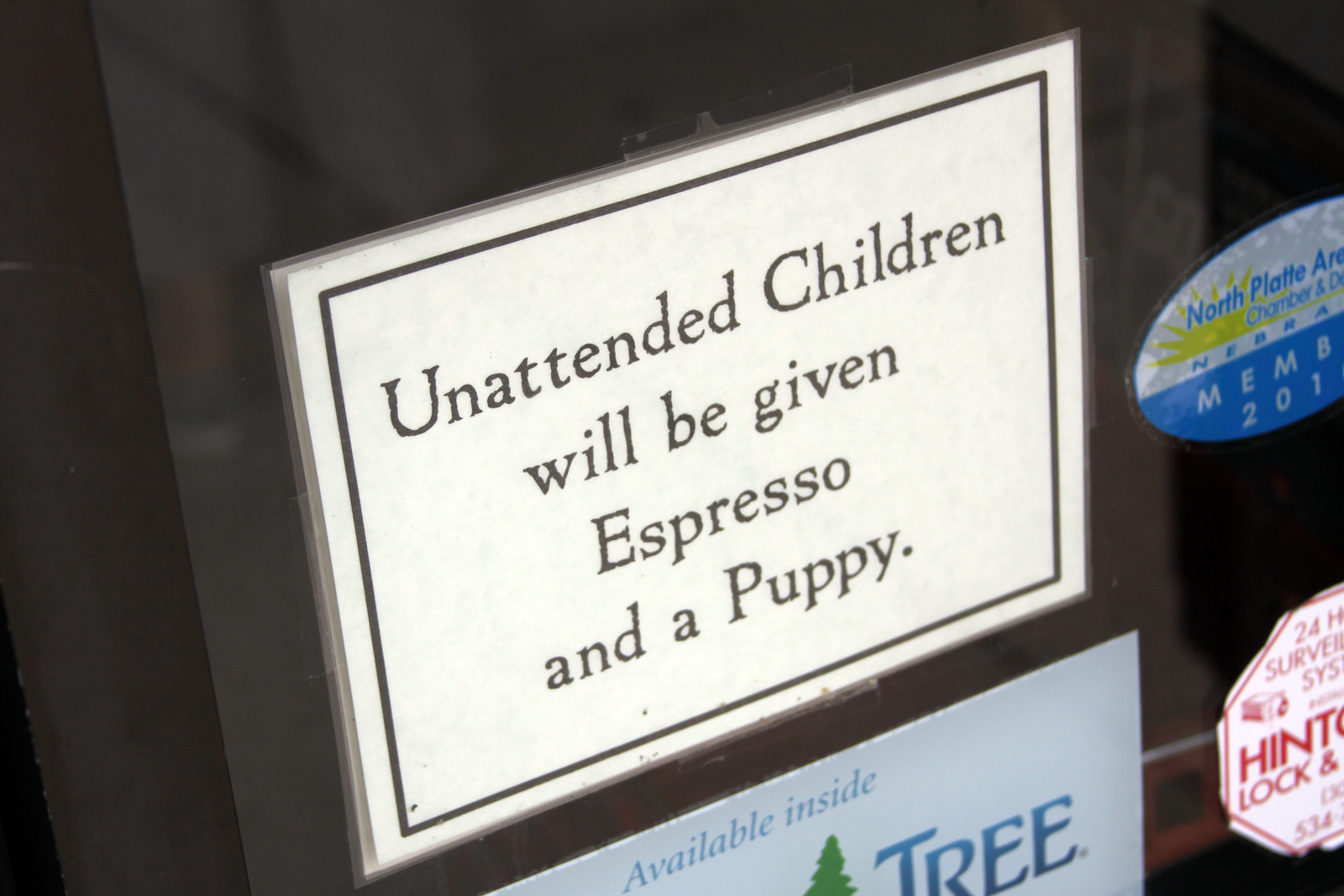The image showcases a laminated white sign, adorned with a thin black border, taped to a glossy black wall that features other stickers. Taken at an angle that makes the right side appear farther than the left, the primary sign bears the bold black text: "Unattended children will be given espresso and a puppy." Below it, another sticker with a white background and blue font reads, "Available inside a picture of a pine tree," followed by the word "tree." On the right side of the sign is a partially obstructed white and blue oval sticker that says, "North Platte Chamber and Nebra Mem 201," though the bottom half is cut off.